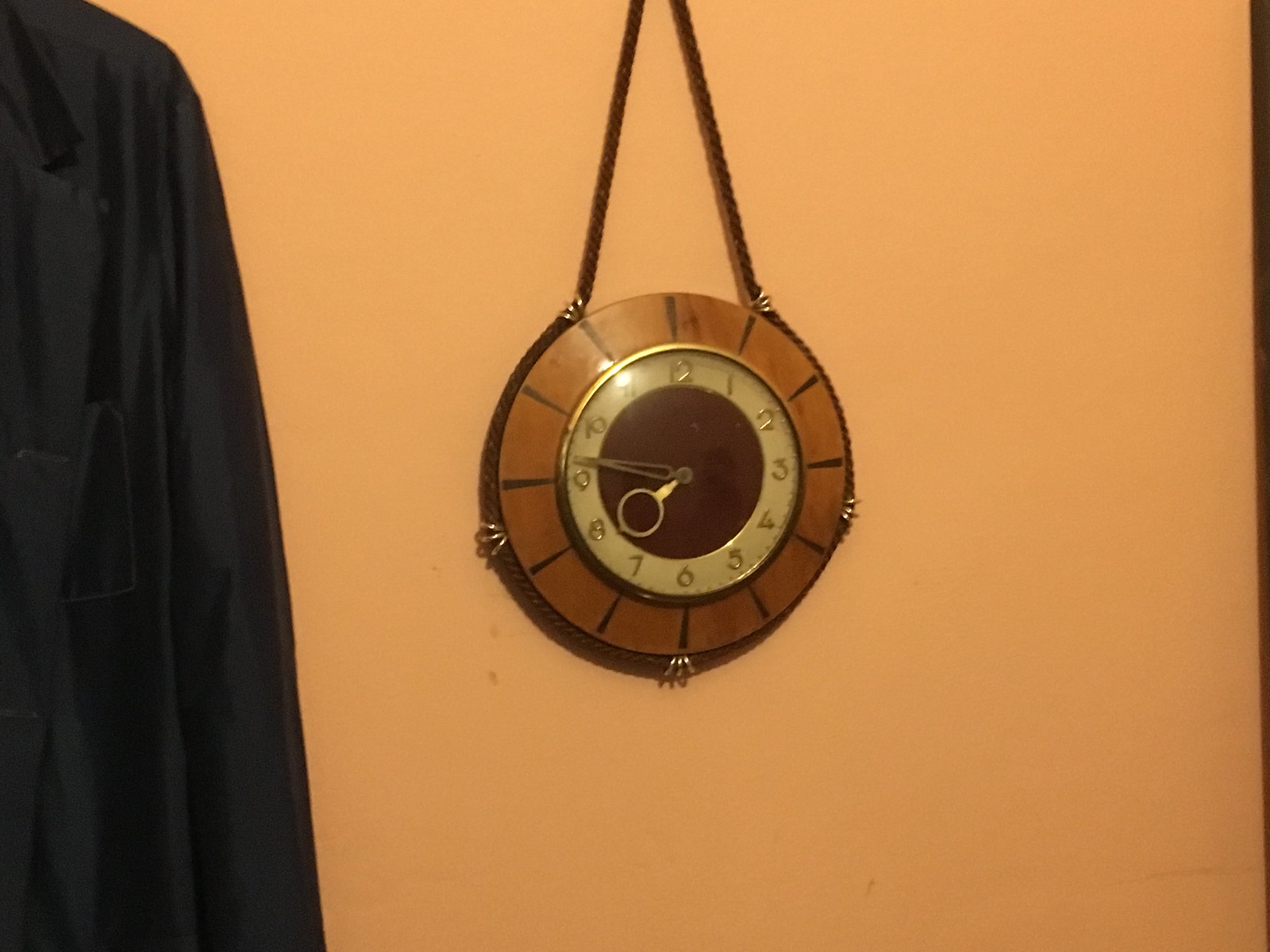The image depicts a vintage or antique-looking clock hanging on a salmon-pink or light peach-colored wall. The clock is circular and designed to be wall-mounted, with a notable design where a brown rope encircles and suspends the clock. This rope threads through five visible clips attached around the outer edge of the clock. The clock face is characterized by gold Arabic numerals marking the hours, from 12 to 12, with black lines under each number. There is a gold ring encompassing the numbers, which themselves are set against a darker brown wooden background. The clock has two distinct hands: the hour hand resembles a pair of tweezers, while the minute hand ends in a circle, designed with a small metal tip indicating the minutes. The current time displayed on the clock is approximately 7:47. Additionally, a black jacket or possibly a men's navy blue suit coat is visible on the left side of the picture, contributing to the overall composition.